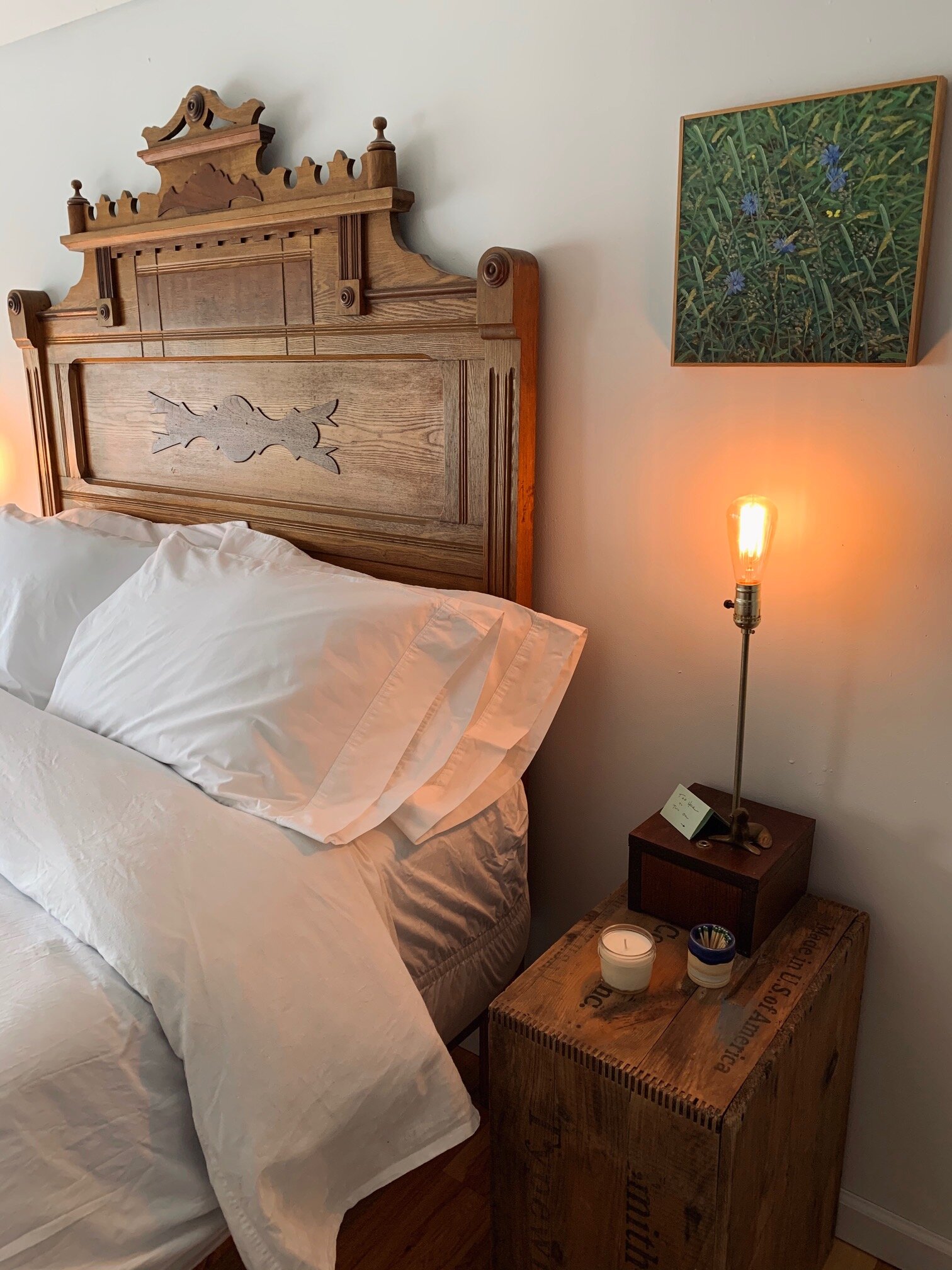This image portrays a photorealistic depiction of a serene bedroom designed with a rustic charm, likely for promotional purposes such as a bed-and-breakfast or Airbnb listing. On the left side, a queen or king-sized bed is adorned with four white pillows, crisp white linens, and a thick, white comforter, all of which face a wooden headboard. This intricately carved headboard features designs reminiscent of chess pieces or castle battlements and possibly an emblem in the center, enhancing the room's vintage feel. 

On the right side of the room, a unique wooden bedside table, crafted to look like an ornate wooden crate complete with braided or interlaced corners, stands next to the bed. Atop this table rests a variety of items: a white candle in a jar, a small cup filled with matches, a small lamp with an exposed retro-style orange bulb, and a box with a note card. Above the lamp, a small photograph depicting blue flowers surrounded by green grasses or weeds is hung on the white wall, adding a touch of nature to the cozy, elegant atmosphere.